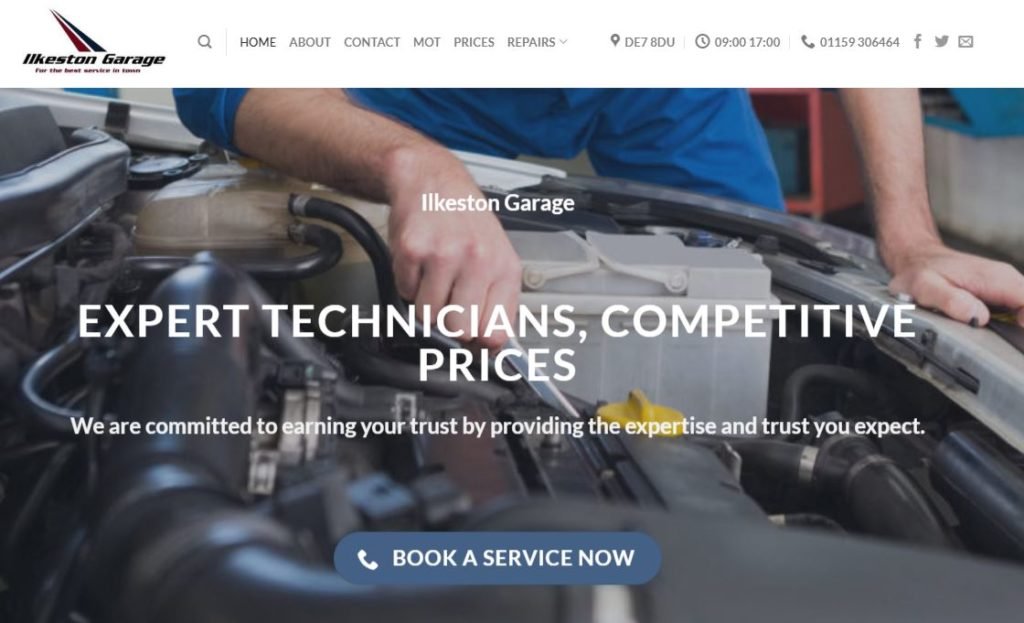The image depicts the homepage of a website titled "Ikeston Garage." At the top, the website's name is displayed prominently with a design that includes small wing-like extensions on either side. The navigation bar includes links labeled "Home," "About," "Contact," "MOT," "Prices," and "Repairs," along with an option to view the garage's location on a map. The website lists operating hours from 9:00 a.m. to 5:00 p.m. and provides a phone number alongside icons for Facebook, Twitter, and email.

A headline reads "Ikeston Garage," followed by the slogans "Expert Technicians" and "Competitive Prices." The text assures customers of the garage's commitment to earning their trust by delivering expertise and reliability.

At the bottom of the webpage, there's a blue, rounded rectangle featuring a white phone icon and the text "Book a Service Now." The background image shows a mechanic, identified as a Caucasian male, working intently on an engine. He is holding a tool and is dressed in a blue shirt with the sleeves rolled up, signaling readiness and professionalism.